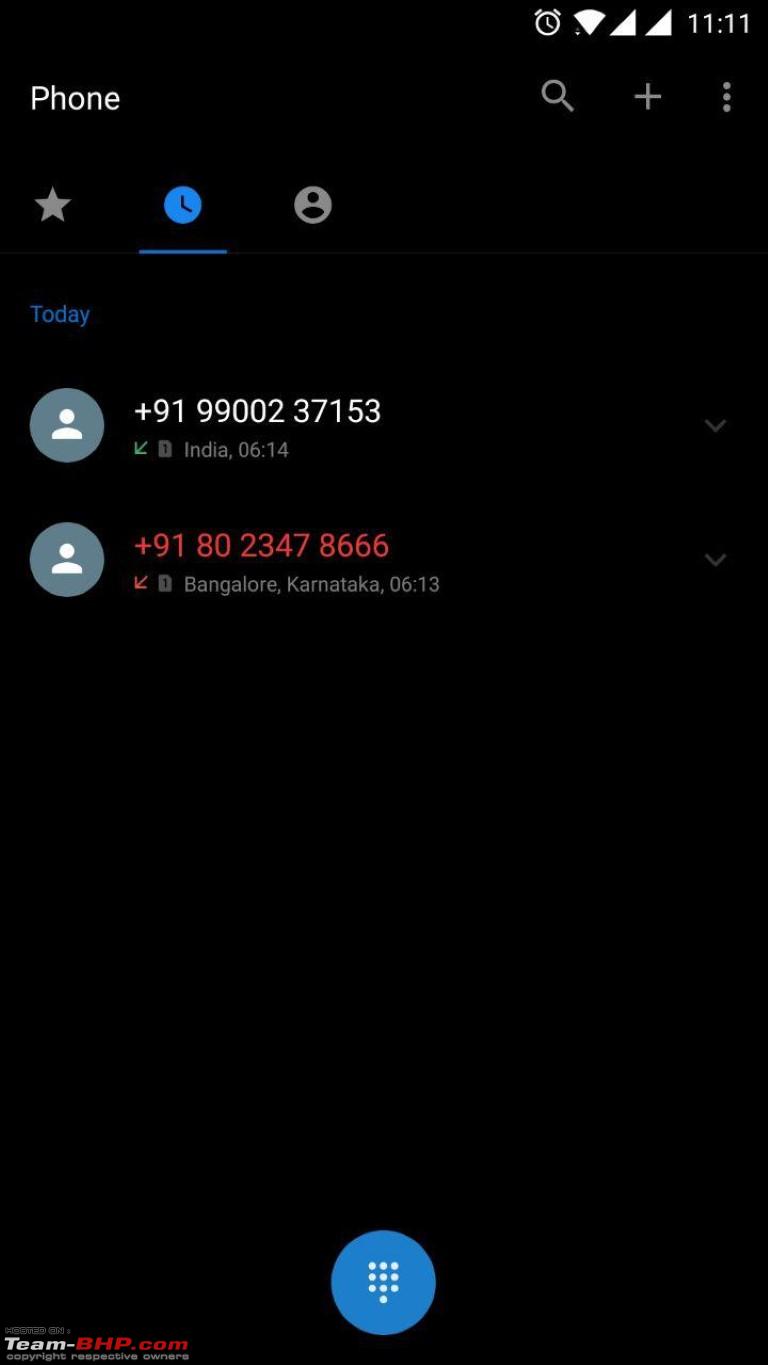The image displays a mobile phone screen in portrait mode with a dark theme. In the top right corner, the status bar features icons for an alarm clock, cellular reception, Wi-Fi, and the current time, which is 11:11. Below the status bar, on the left side, the word "Phone" appears in white text. To the right of this, there are several gray icons including a magnifying glass, a plus sign, and three vertical dots.

Further down, there's a section with a gray star, a blue clock icon which is underlined, and a gray profile icon. Below this section, the word "Today" is shown in blue text next to another gray profile icon, followed by an Indian phone number: "+91 9900237153". Underneath the phone number, it displays an arrow with the number "1" beside it, the label "India," and the time "06:14".

Beneath this, another phone number is displayed: "+91 8023458666" with the label "Bangalore Karnataka" and the time "06:13". At the bottom of the screen, there is a round blue button featuring white dots forming an arrow, and on the bottom left corner, "team-bhp.com" is indicated.